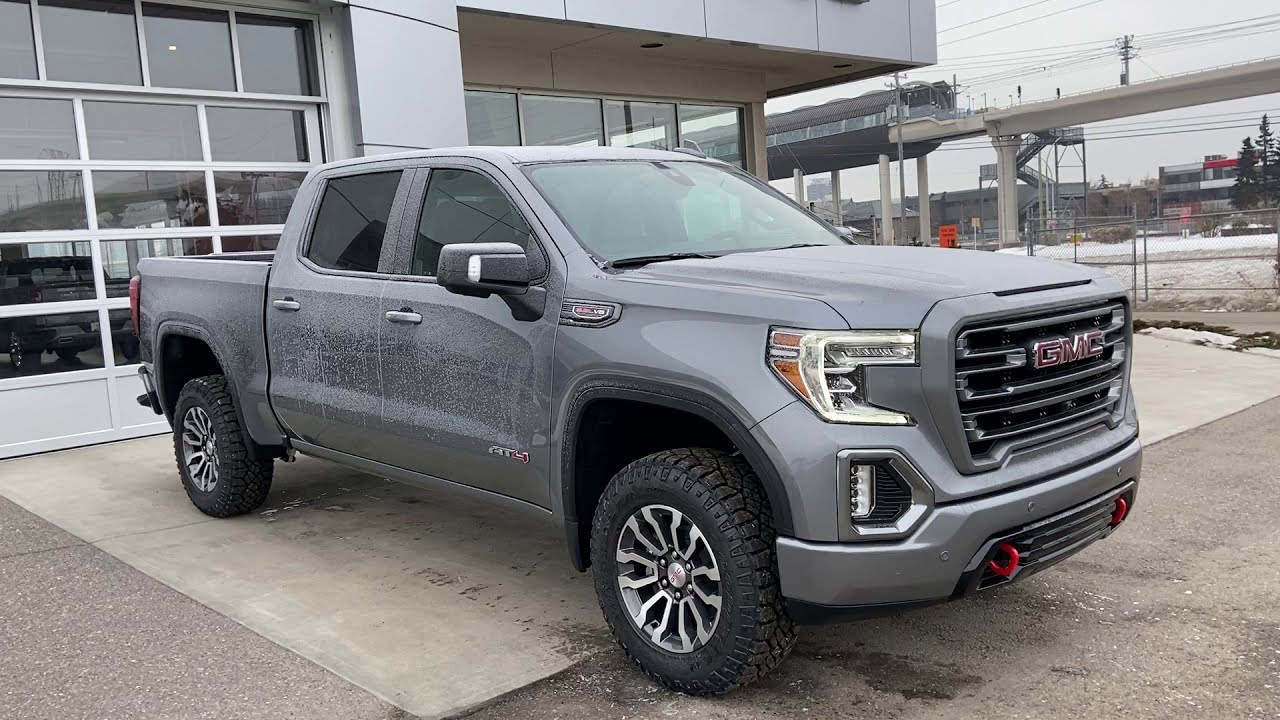In this daytime photograph, the central focus is a diagonally parked, dark gray or silver GMC Sierra pickup truck occupying the middle of what appears to be an asphalt parking lot outside a car dealership. The truck’s grill prominently features large, red "GMC" letters flanked by two red pole bars. The truck is slightly dirty, with white markings on the sides suggestive of previous snow or rain exposure. Its clean, shiny silver rims and large, raised snow tires hint at rugged utility. Behind the truck, there's a steel-paneled building with a large garage door embedded with windows, through which another truck is visible. To the right side of the image, a gate, power lines, and a large elevated structure resembling a monorail track or bridge underscore the setting, providing an industrial feel. The color palette of the scene includes shades of gray, black, silver, yellow, red, white, light blue, and orange, depicting a dynamic and detailed outdoor environment.